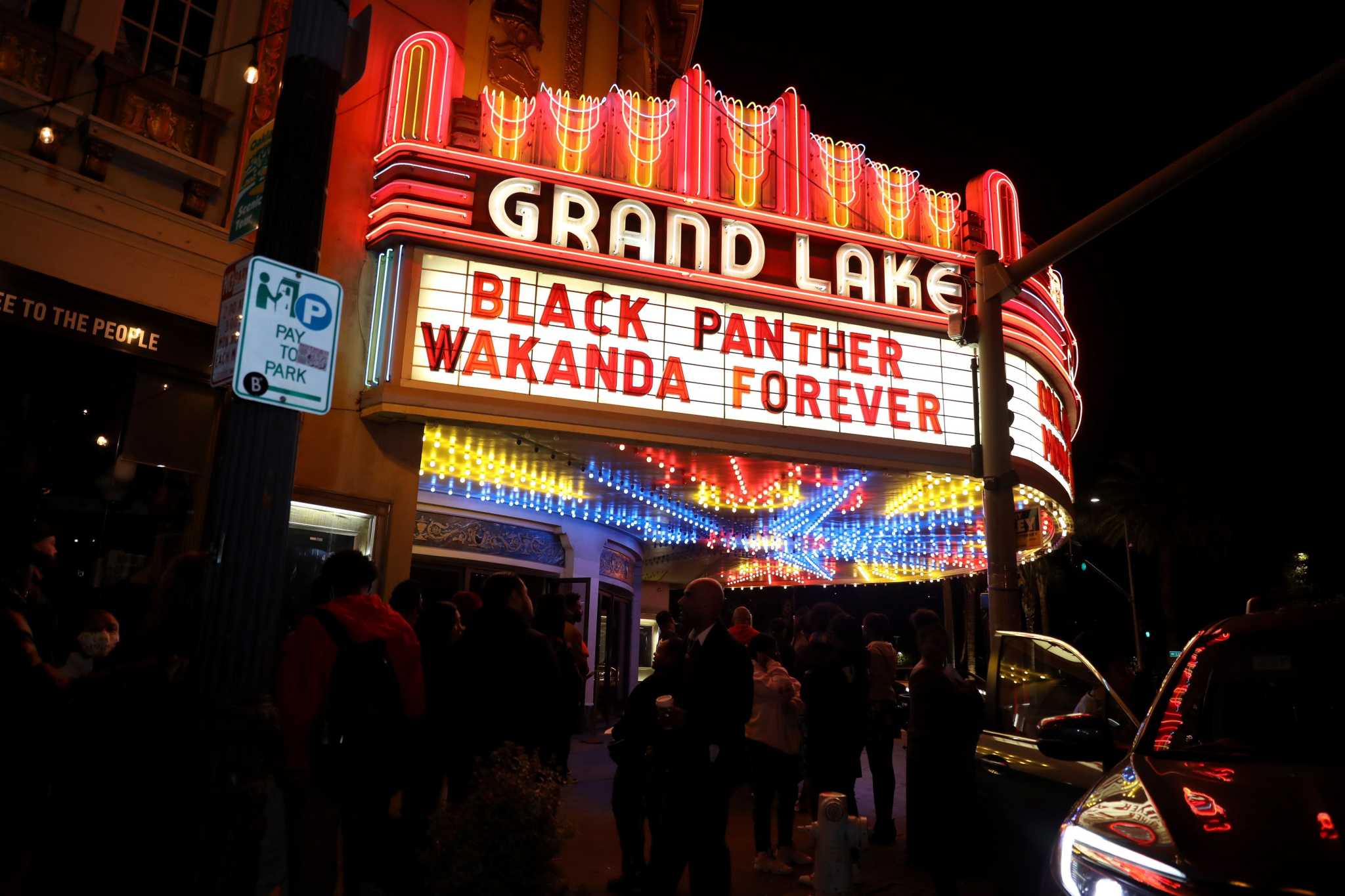The image captures a nighttime scene outside the highly illuminated Grand Lake Theater. Dominating the composition is the theater's grandiose marquee, adorned with striking neon lights in red, yellow, and orange, culminating in an elegant display. In bold, white capital letters against a black background, the marquee proudly proclaims the theater's name, Grand Lake. Below, a vibrant sign announces the evening's feature film, "Black Panther: Wakanda Forever," written in vivid red letters on a clean white backdrop. The marquee extends outward, casting a colored glow of red, yellow, and blue lights that enhances its captivating appeal.

Beneath this luminous sign, a small crowd of people is gathered, waiting in the shadows to enter the theater. The scene includes additional details, such as a "Pay to Park" street sign visible on the left side of the image, heightening the sense of the theater's bustling urban locale. To the right, partially under the marquee, the front of a car with its door open reflects the theater’s lights, adding depth and context to the nocturnal setting. Though the background is dark and other structures are obscured, the detailed focus on the theater's marquee creates a dramatic and vivid portrayal of the scene.